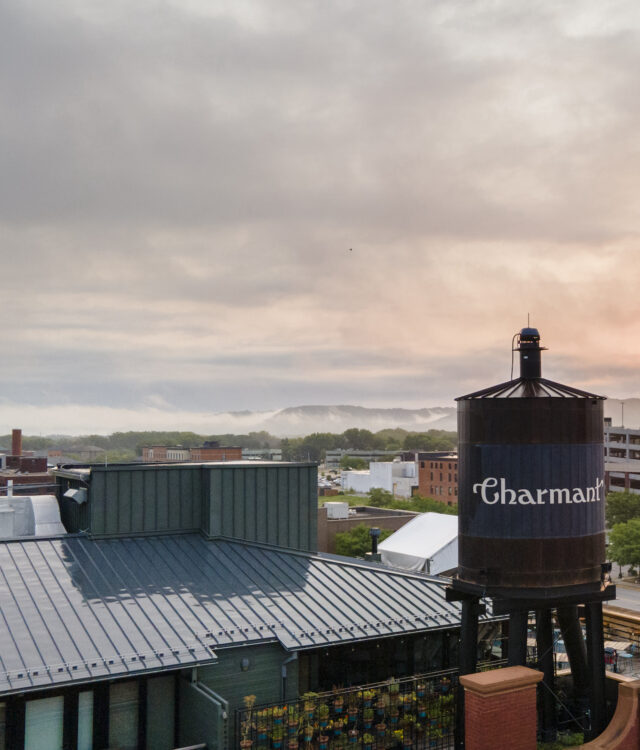The image captures the back of a building, focusing primarily on its dark green metal roof. To the right of the roof stands a water tank labeled "Charmant." The scene is set against a dark, cloudy sky, with part of a mountain visible to the left of the water tank. Trees and various other buildings populate the background, contributing to the small-town skyline feel. In the bottom right corner of the photo, there is a brick column next to which a wall adorned with several potted plants is visible. The foreground also includes a section that seems to be a patio area, featuring tables with tablecloths and chairs, enclosed by a wooden wall. Scattered industrial and brick buildings, along with a faint glimpse of a street, hint at a mixed-use area. The overall atmosphere is under a thick cloud cover, enhancing the moody, overcast ambiance.